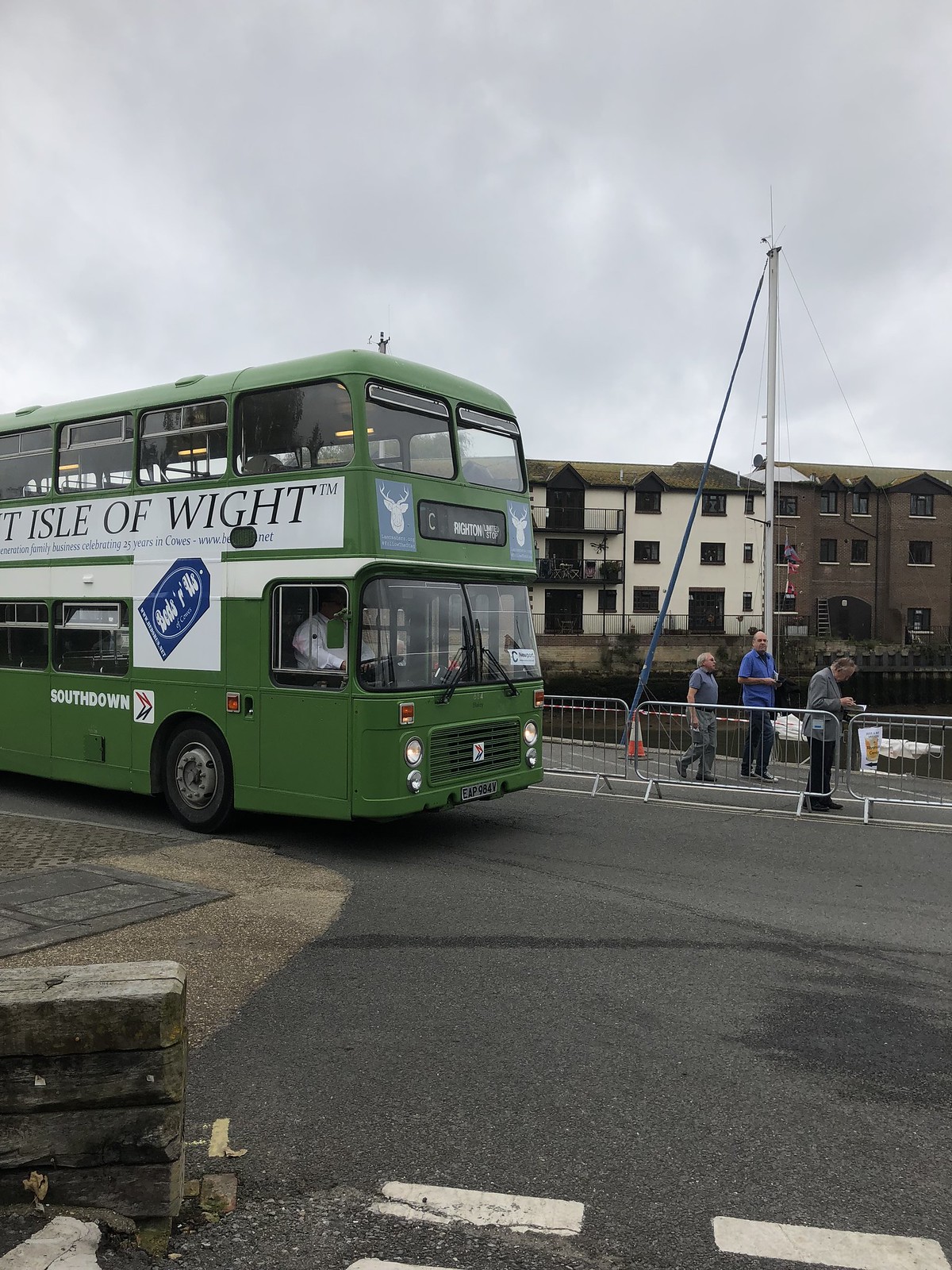This photograph showcases a green, two-story double-decker tour bus entering the frame from the left side. The bus is dark green with two blue squares with white logos, featuring deer, on its front. Positioned roughly at a 330-degree angle, it appears to be in motion down the middle of a street. The front half of the bus is visible, with "Isle of Wight" inscribed in black text on a white banner along its side, indicating its destination. The driver can be seen through the front window, and the bus is illuminated from within. In the background, the scene is set against an overcast sky with a gray, cloudy atmosphere. To the right of the bus, three elderly men walk along a fenced sidewalk, which runs parallel to a body of water. Visible in the water is the mast of a sailboat, and behind it, two apartment buildings—one ivory and one brown—feature balconies facing the scene. The combination of the tour bus and the surrounding urban environment with water and buildings gives the impression of a bustling, albeit overcast, day in a scenic locale.